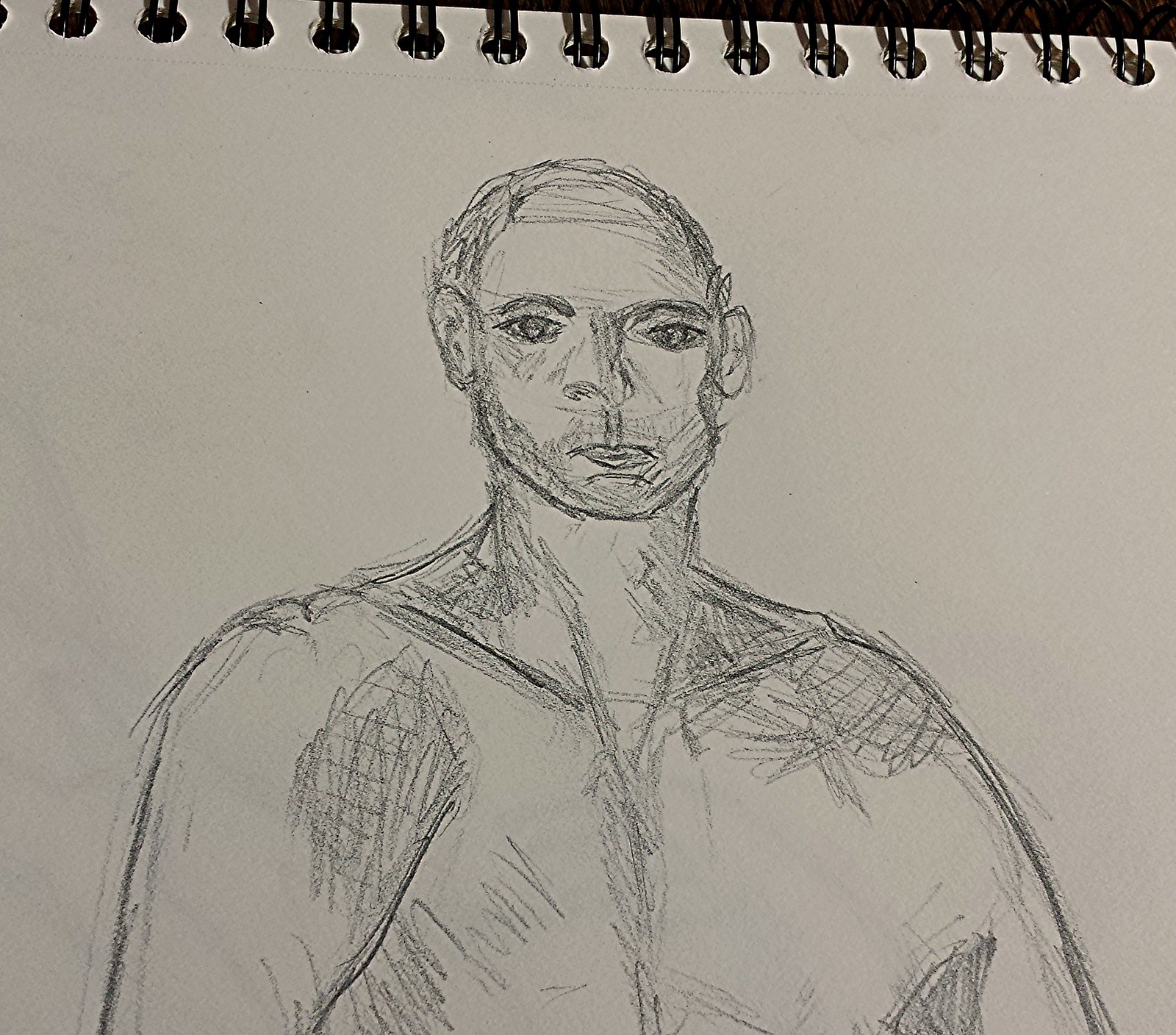This close-up photograph captures the entirety of a sketchbook, filling the frame from edge to edge with no discernible background. Dominating the upper part of the image is the spiral binding, indicating the top of the notebook. The blank sketchbook page, an expanse of unmarked white paper, features a pencil sketch of a man. The man's gaze is fixed directly at the viewer, donning a neutral expression that conveys neither happiness nor distress. The intricate pencil work showcases areas of shading, meticulously rendered with a grid pattern to create depth and texture.